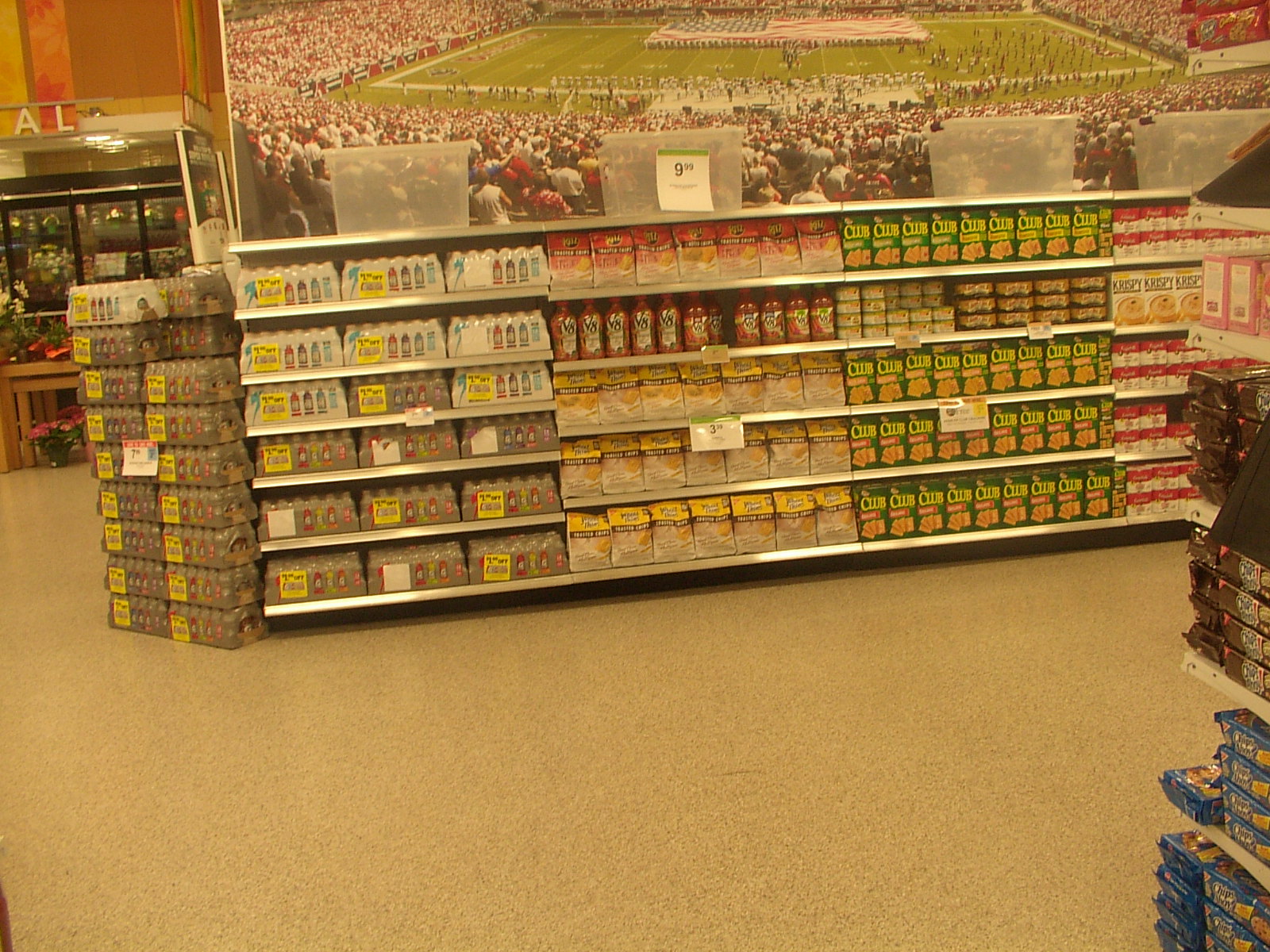In this vibrant supermarket scene, the camera captures the bustling interior of an aisle laden with various products. Centrally displayed are stacks of goods, possibly boxes of crackers and an assortment of snacks, meticulously arranged to draw shoppers' attention. Nearby are numerous drinks, prominently featuring V8 beverages, with bold signage indicating prices in close proximity — a notable sign displays "$9.99," though it is ambiguous whether this price pertains to the bags of snacks or the V8 drinks beneath it. Adding to the atmosphere, a striking mural depicting a football field serves as an engaging backdrop, seamlessly blending the themes of food and sport within the shopping environment.